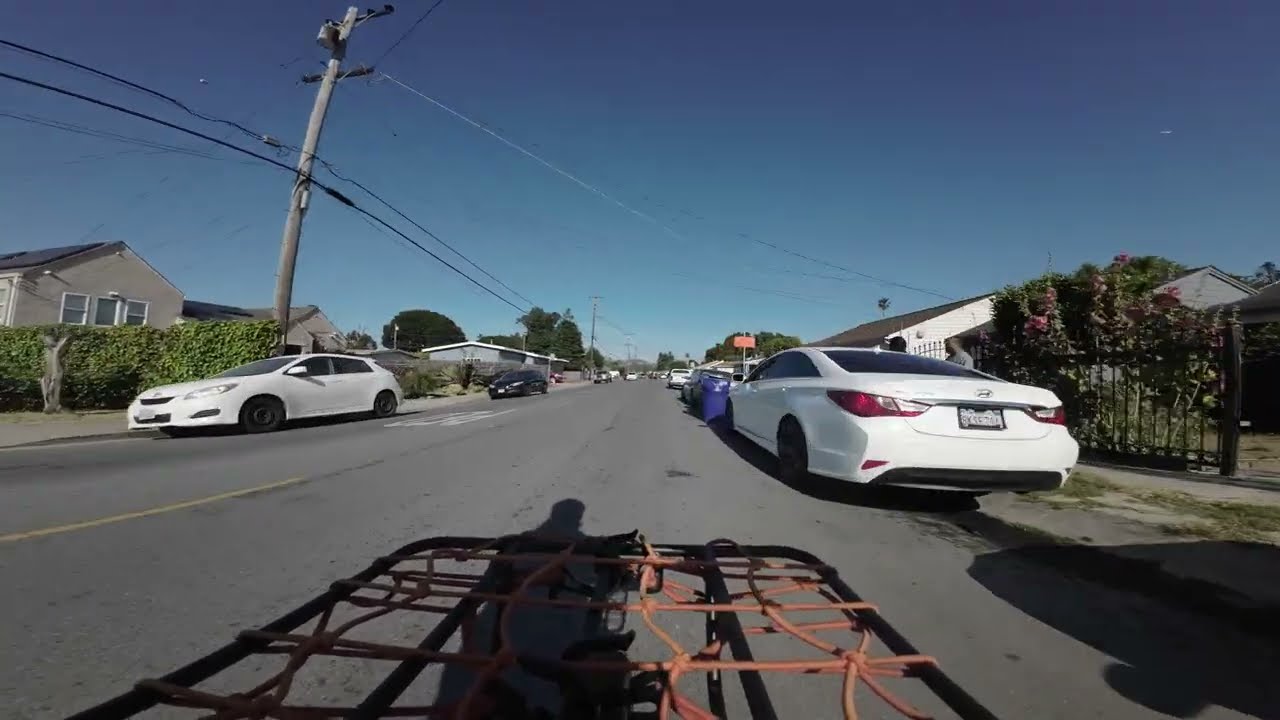In this fisheye-lens image, we see a suburban street scene from the perspective of someone possibly pushing a cart or riding a bicycle equipped with a black metal frame and bungee cords for storage. The shadow of the person falls slightly to the left of the frame. The street itself is a typical blacktop road with yellow lines down the center and gray cement sidewalks on either side. Cars are parked along both sides of the road: those on the right are facing forward, while those on the left are facing toward the viewer. Residential houses line the street, featuring a mix of tan and white facades, with fences, walls, and large green shrubs. Pink flowers climb one of the fences. In the foreground, there's a white Hyundai sedan with a blue trash can in front of it. Further down the street, a pole with a sign is visible. Two people can be seen talking near the car on the right side. The setting appears to be early evening under a clear blue sky, with distant hills suggesting a Southern California locale.